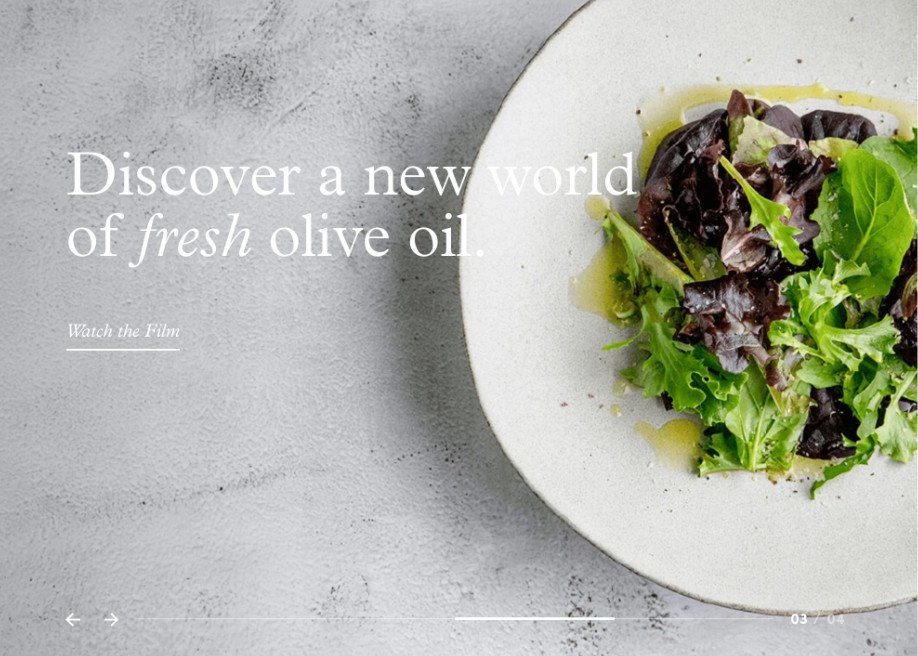The image features a beautifully crafted website layout set against a distressed light gray background with darker gray accents, giving a textured and rustic feel. Dominating the center is a stunning, high-resolution photograph of a sophisticated salad displayed in a dish with a grayish trim. The salad is composed of fresh spring garden greens, delicately grated cheese, and a drizzle of premium olive oil romantically spread over and around the greens. 

Above the dish, bold white letters invite the viewer to "Discover a new world of fresh," with "fresh" stylized in a fancy font. Below this enticing tagline, a blue hyperlink underlined in white prompts users to "Watch the film." 

Positioned at the lower corners of the image are navigation arrows and a pagination indicator, showing "3 of 4" in the lower right. The overall presentation subtly suggests that the olive oil used as a dressing is of exceptional quality, appealing to those seeking a refined culinary experience.